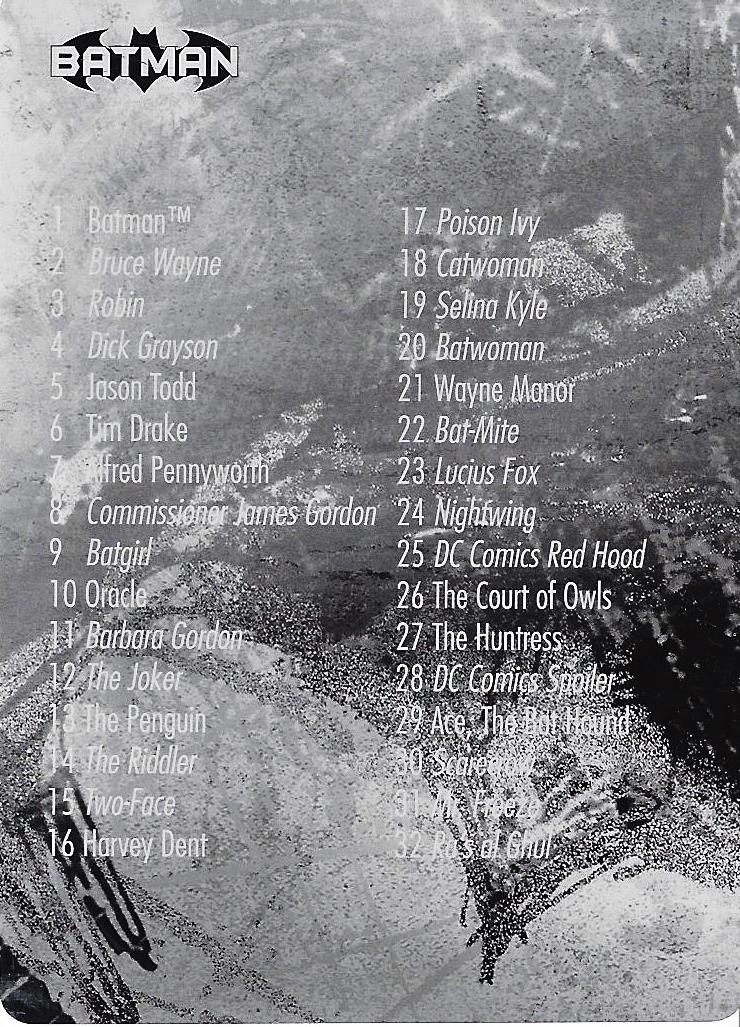The image features a grungy, artsy background with a predominantly gray and black palette, characterized by scratchy, streaked patterns and flecks of white, resembling a faded, concrete surface. In the upper left corner, there is a black Batman logo with the word "BATMAN" written over it in capital white letters. The background is overlaid with white text forming a list of 32 comic book characters. The numbered list runs from 1 to 16 on the left and 17 to 32 on the right. The first 16 entries are: 1. Batman, 2. Bruce Wayne, 3. Robin, 4. Dick Grayson, 5. Jason Todd, 6. Tim Drake, 7. Alfred Pennyworth, 8. Commissioner James Gordon, 9. Batgirl, 10. Oracle, 11. Barbara Gordon, 12. The Joker, 13. The Penguin, 14. The Riddler, 15. Two-Face, and 16. Harvey Dent. The remaining entries from 17 to 32 are: 17. Poison Ivy, 18. Catwoman, 19. Selina Kyle, 20. Batwoman, 21. Wayne Manor, 22. Batmite, 23. Lucius Fox, 24. Nightwing, 25. Red Hood, 26. The Court of Owls, 27. The Huntress, 28. Spoiler, 29. Ace the Bat Hound, 30. Scarecrow, 31. Mr. Freeze, and 32. Ra's Al Ghul.